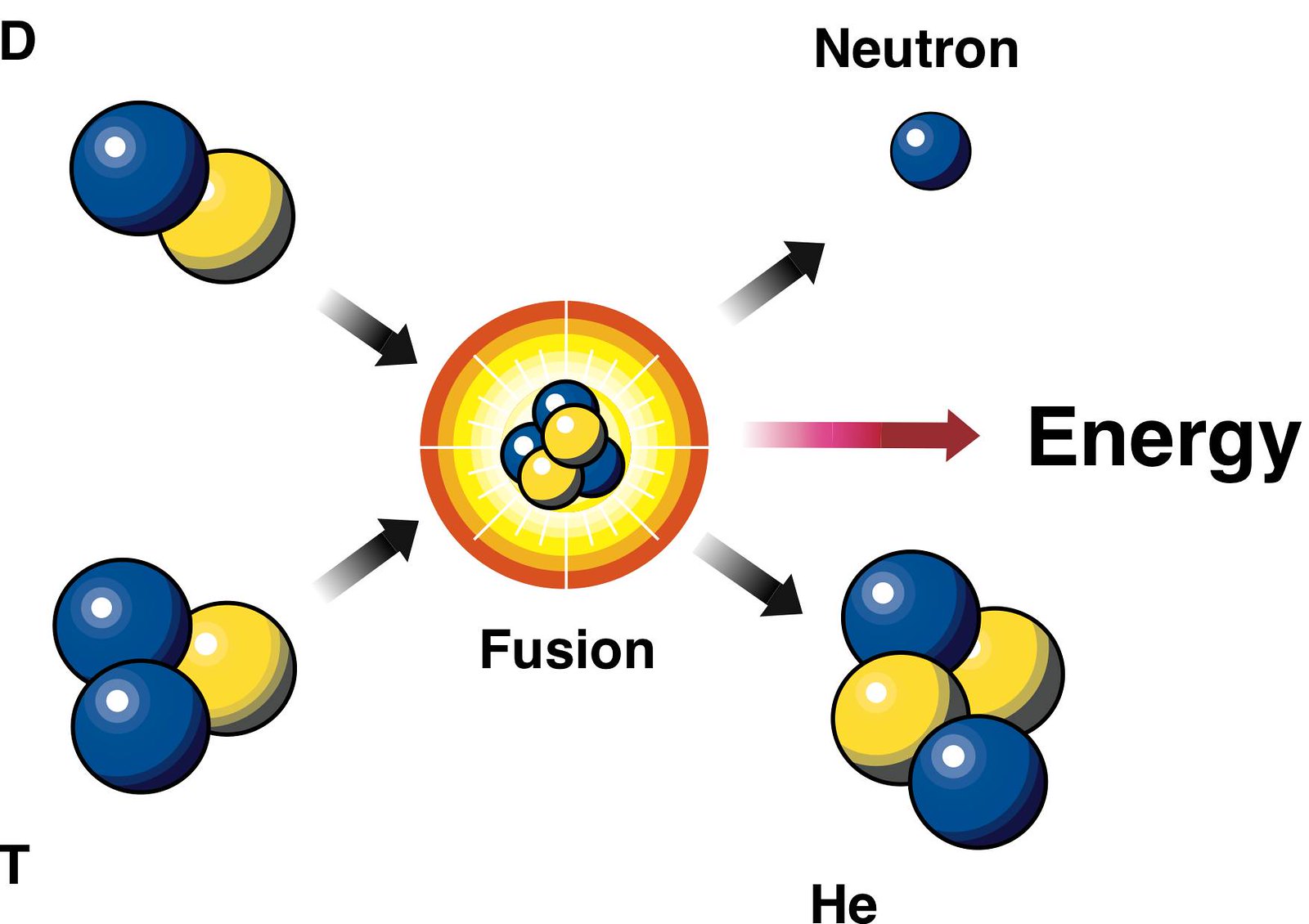The image is a detailed piece of graphic art depicting an atom represented by a cluster of yellow and blue spheres, surrounded by concentric rings in white, yellow, orange, and red. From the top left, the letter "D" is labeled, featuring a blue sphere over a yellow sphere, with a black arrow pointing at the atom. In the lower left, the letter "T" is illustrated with two blue spheres and one yellow sphere, also marked by a black arrow pointing at the atom. The top right section shows the word "Neutron" with a single blue sphere and a black arrow pointing at it. The middle right side is labeled "Energy," with a red arrow indicating the word. At the bottom right, the image features the word "He" with two blue spheres and two yellow spheres, accompanied by a black arrow pointing toward them. The background is white, and the diagram includes a total of five arrows—four black and one red—adding to the intricate layout of the scientific illustration.